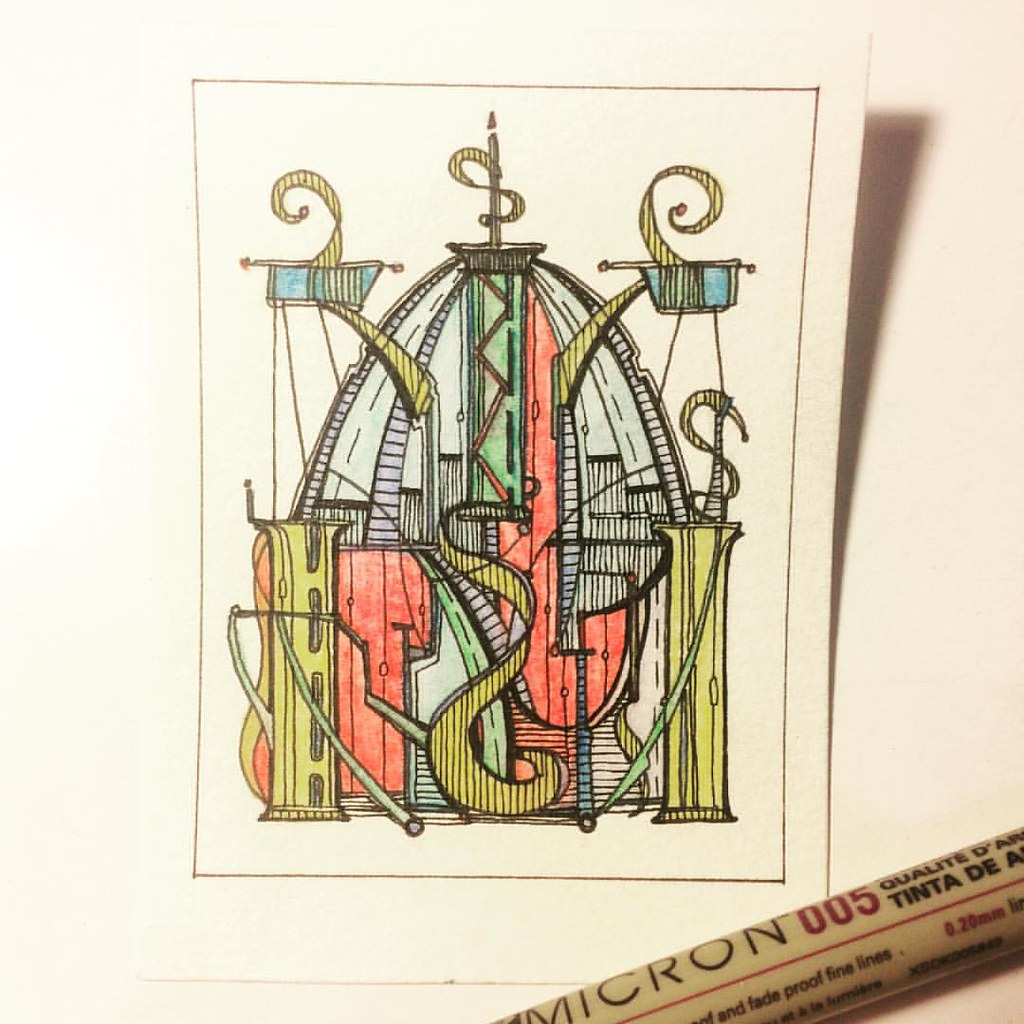This is a photograph of a small, intricate piece of abstract art captured in portrait mode. The image includes a pen, labeled "Micron 005 Qualite Tinta De" with a fine red line and "fade proof fine lines" text, stretching from the center left to the bottom right, providing scale and emphasizing the diminutive size of the artwork. The drawing features a complex, abstract design with an array of colors such as yellows, oranges, blues, and greens. The artwork itself is on a cream-colored background, with the drawing forming an almost dome or egg shape, filled with curved roads, spiral staircases, and other whimsical, musical note-like shapes. There are intricate yellow tubes on the sides, red curves, and various other detailed elements that lend it a modern art feel. At the top of the image, the design curves, and some elements resemble small cups, adding to the overall artistic and modern aesthetic of the piece.